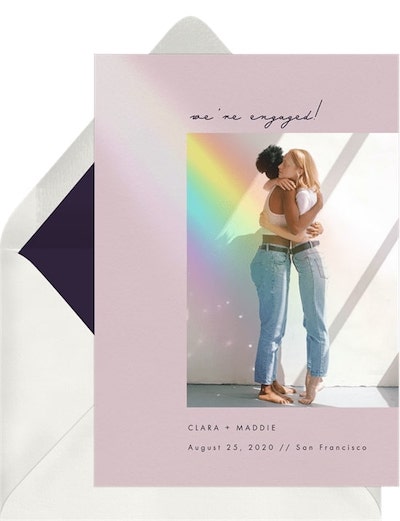The photograph features an engagement announcement on a piece of paper, with an opened white envelope behind it. The background of the announcement is a purplish-pink hue. At the top of the announcement, in a cursive script, it reads "We're engaged!" with an exclamation point. Below this, there is an image insert showing two women embracing intimately. Both women are barefoot and dressed similarly in light-washed denim jeans with black belts and white tops—one in a t-shirt and the other in a tank top. The woman with blonde hair, who appears to be white, stands on her tiptoes with her profile more visible, while the woman with dark hair, who appears to be African-American, embraces her. The text below the image reads "Claire M. Medin." The date of the engagement is noted as August 25, 2020, with the event set to take place in San Francisco. A faint, semi-transparent rainbow arcs from the top left toward the center, adding a whimsical touch. The lighting in the indoor photograph highlights the embracing couple, coming from the right corner and illuminating the scene beautifully.